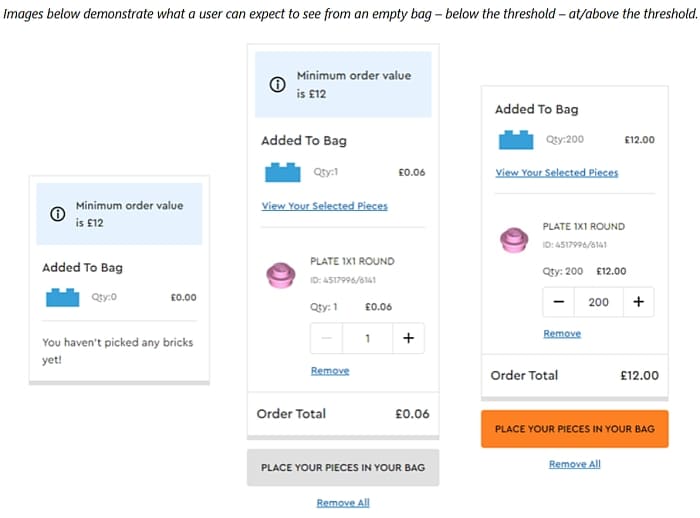This image consists of a screenshot with a white background, featuring a series of items displayed in three distinct sections, each representing different states of a user's shopping experience relative to a defined threshold. 

At the very top, there is a single line of black text stating: "Images below demonstrate what a user can expect to see from an empty bag, below the threshold, at/above the threshold." 

Below this line, there are three visual representations arranged horizontally:

### Left Section (Empty Bag)
- **Layout**: A square shorter than the other two sections.
- **Top**: A blue rectangle with a black circular icon containing a lowercase 'i' on the left. Beside the icon, in black text: "Minimum order value".
- **Price**: Two lines below, in black text: "£12".
- **Main Content**: In bold black text within another blue rectangle: "Added to bag". 
- **Quantity and Price**: To the right of this, in gray text: "qty: 0". In bold black beside it: "£0.00". This is underlined by a light gray line.
- **Message**: Below the underlined section, in black text: "You haven't picked any bricks yet!"

### Middle Section (Below Threshold)
- **Layout**: A taller rectangle.
- **Top**: Similar blue rectangle and circular icon as the left section.
- **Price**: Black text stating: "£12".
- **Main Content**: Bolded black text: "Added to bag".
- **Quantity and Price**: Gray text: "qty: 1". In bold black beside it: "£0.06". Underlined by a light gray line.
- **Link**: Below this, a clickable underlined link in light gray: "View your selected pieces".
- **Item Details**: Displays a pink tall plate with two bowls stacked on plates to the right. Item is described as "plate txt round" with an ID number and black text: "Quantity: 1". Price: "£0.06".
- **Adjust Quantity**: A rectangle split into three sections with a gray minus sign on the left, a black number '1' in the center, and a black plus sign on the right.
- **Link**: An underlined "Remove" link in blue.
- **Total**: Bolded black text: "Order total: £0.06".
- **Button**: A gray rectangular button: "Place your pieces in your bag".
- **Remove All**: Below this button, an underlined text: "Remove all".

### Right Section (At/Above Threshold)
- **Layout**: A rectangle shorter than the middle one.
- **Top**: Similar blue rectangle and circular icon as the other sections.
- **Price**: Black text: "£12".
- **Main Content**: Bolded black text: "Added to bag".
- **Quantity and Price**: Gray text: "qty: 200". In bold black beside it: "£12.00". This is underlined by a light gray line.
- **Content Below**: Not described in detail, but set up similarly to the middle section with applicable adjustments for higher quantity.

Each section provides a clear visualization of the shopping cart status at different stages: empty, below the threshold, and meeting/exceeding the order threshold.